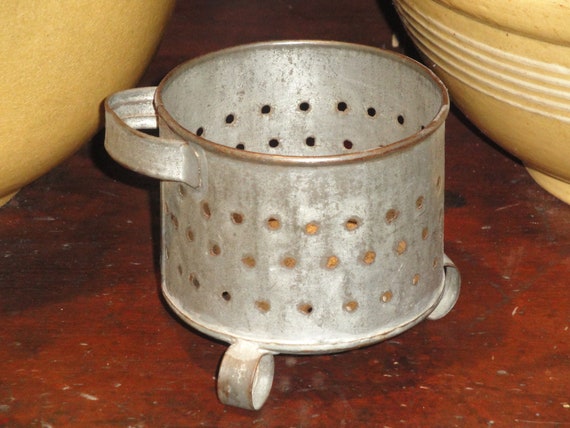This image captures a detailed close-up of a rustic setting featuring an old, metal sifter at the center. The sifter, made of tin and featuring a bronze ring around the top, has three levels of holes and small round feet. It’s equipped with a curved handle on the left side and shows signs of wear. Flanking the sifter on both sides are two orangish-yellow ceramic bowls, though only partial views of them are visible. The bowl on the left is a solid color, while the one on the right has five white stripes around it. These items are placed on a maroon, possibly dirty and streaked countertop or table, which has various splotches of white. The combination of the old sifter and the ceramic bowls sets a vintage ambiance, suggesting a kitchen setting preparing for baking or some agricultural task.